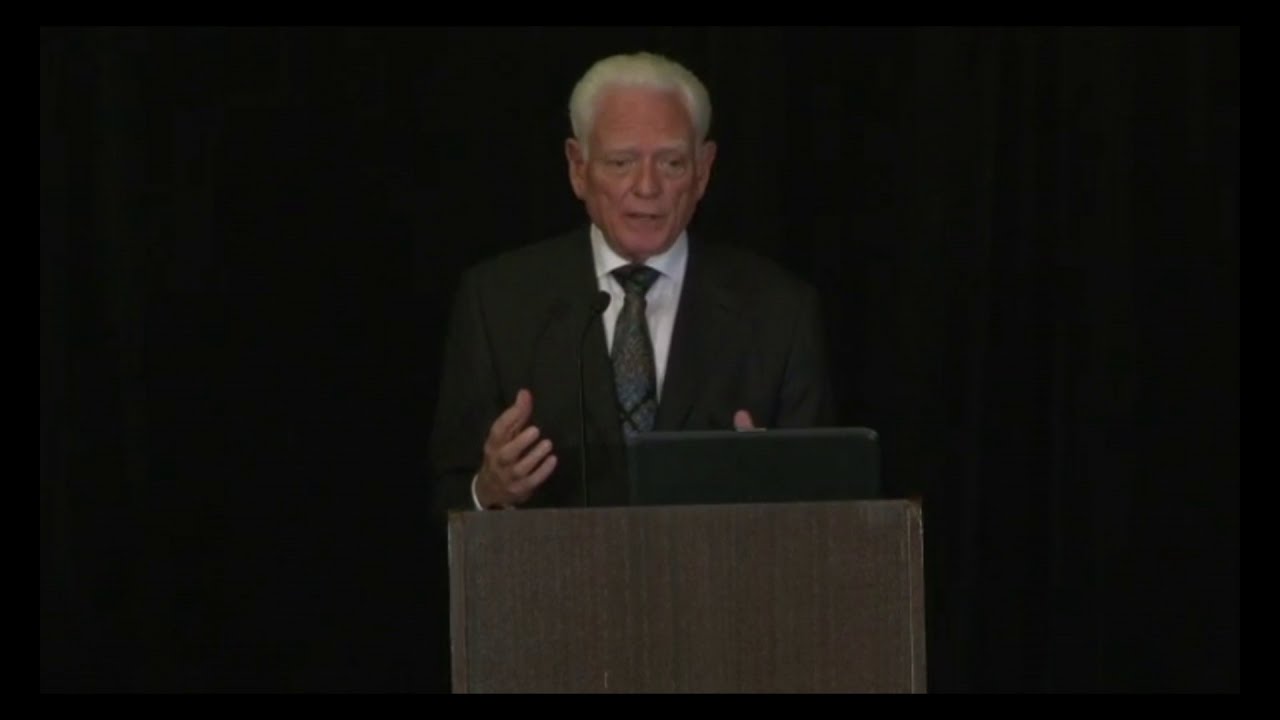The image depicts an elderly gentleman, likely in his 80s, standing behind a worn brown podium, possibly giving a speech or a sermon. He is dressed in a black suit with a white dress shirt and a dark, possibly grayish-black, tie adorned with an X pattern. His stark white hair contrasts against the black drapery backdrop, making him more noticeable. He gestures with his hands, emphasizing his points during the talk. A thin black microphone is attached to the front of the podium, blending somewhat with his suit jacket. Additionally, there appears to be a laptop or tablet on the podium, suggesting he might be using it for his presentation. His prominent white eyebrows and large ears add to his distinguished appearance. The setting and composition suggest that this might be a still from a video recording of his presentation.